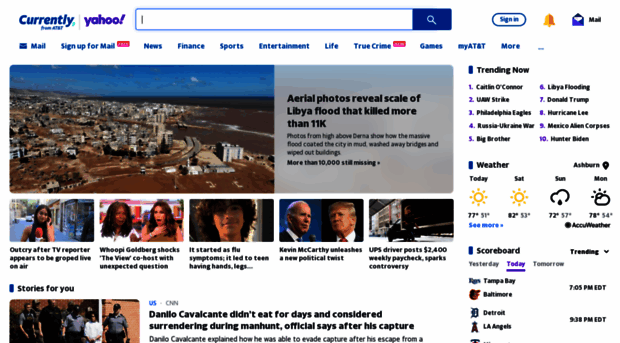Here is a cleaned-up and detailed caption for the image described:

---

The splash screen of Yahoo.com is prominently displayed against a white background, exuding a bustling and vibrant appearance. At the upper left corner, the word "Currently" is stylishly italicized in blue font, accompanied by additional text beneath it. To its right, the iconic purple Yahoo! logo with an exclamation mark stands out. Centrally positioned near the top, a white search box invites users to enter their search terms, featuring a magnifying glass icon with a blue background. Adjacent to this search box are icons for signing in, a bell notification, and an envelope labeled "Mail".

Dominating the left-central portion of the screen is an aerial photograph of a city bathed in clear blue skies. To the right of this image, a sobering headline reads, "Aerial photos reveal scale of Libya flood that killed more than 11k," with a further description below it. In a darker font beneath the description, it somberly states, "More than 10,000 still missing."

On the right side of the screen, a section titled "Trending Now" lists the top 10 trending topics, with "Caitlyn O'Connor" leading the list. Below this is the weather section, showcasing sunny icons for today and Saturday, a cloud with a raindrop icon for Sunday, and a mix of cloud and sun icons for Monday.

Further down is the "Scoreboard" section, highlighting ongoing games including Tampa Bay vs. Baltimore and Detroit vs. Los Angeles. In the bottom-left of the image, a segment titled "Stories for You" is marked by a blue rectangle. This section includes a photograph of police officers escorting a handcuffed individual. To the right of this image, the headline in bold black font reads, "Danilo Cavalcante didn't eat for days and considered surrendering during the hunt, officials say, after his capture."

---

This enriched caption provides a thorough and visually descriptive summary of the splash screen, conveying key details for a reader.